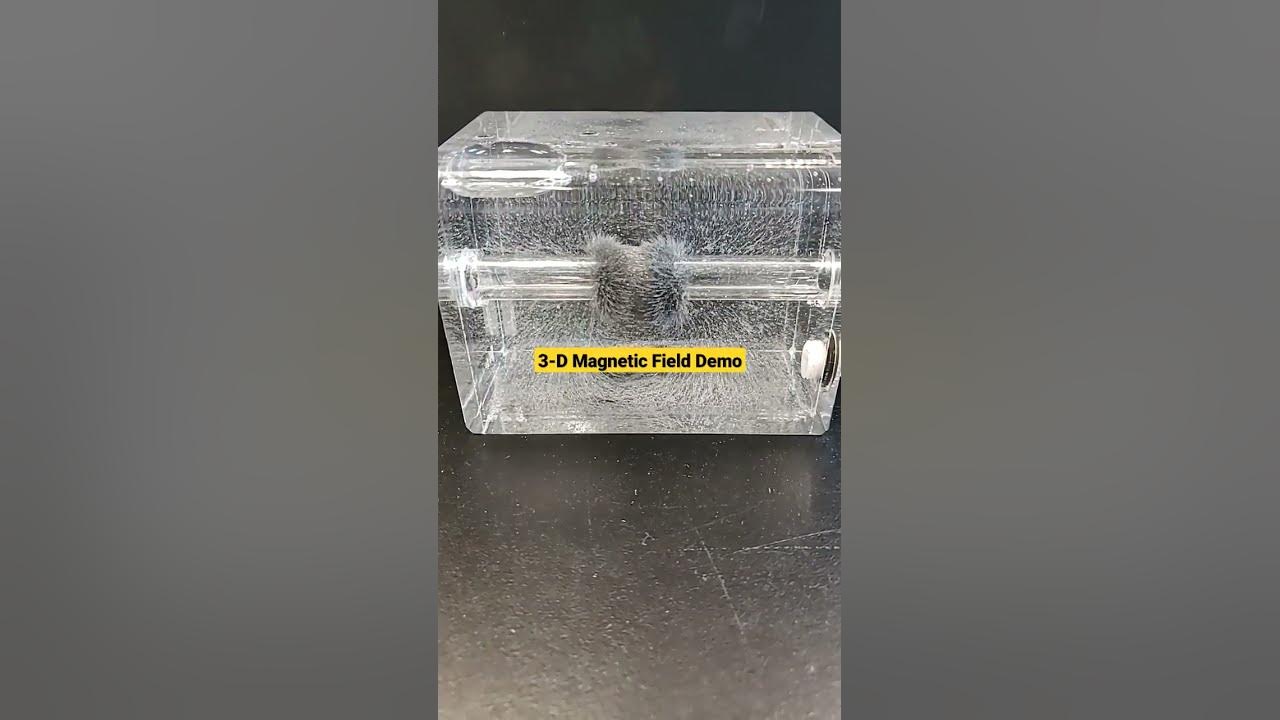This black and white image showcases an intricate 3D Magnetic Field Demo displayed inside a transparent, cube-shaped container. A yellow rectangular label with black sans serif font reading "3-D Magnetic Field Demo" is prominently featured on the front face of the cube. Inside the cube, a centrally-placed cylinder is densely packed with clustered gray material, possibly representing magnetic bits or wires that demonstrate magnetic field properties. Notably, a bar or handle runs along the side of the container, contributing to its three-dimensional structure. At the bottom right within the cube, a distinctive white disk or plug stands out, resting on a dark black surface. This setup is flanked by significant gray panels on either side, adding to the overall context of the demonstration.